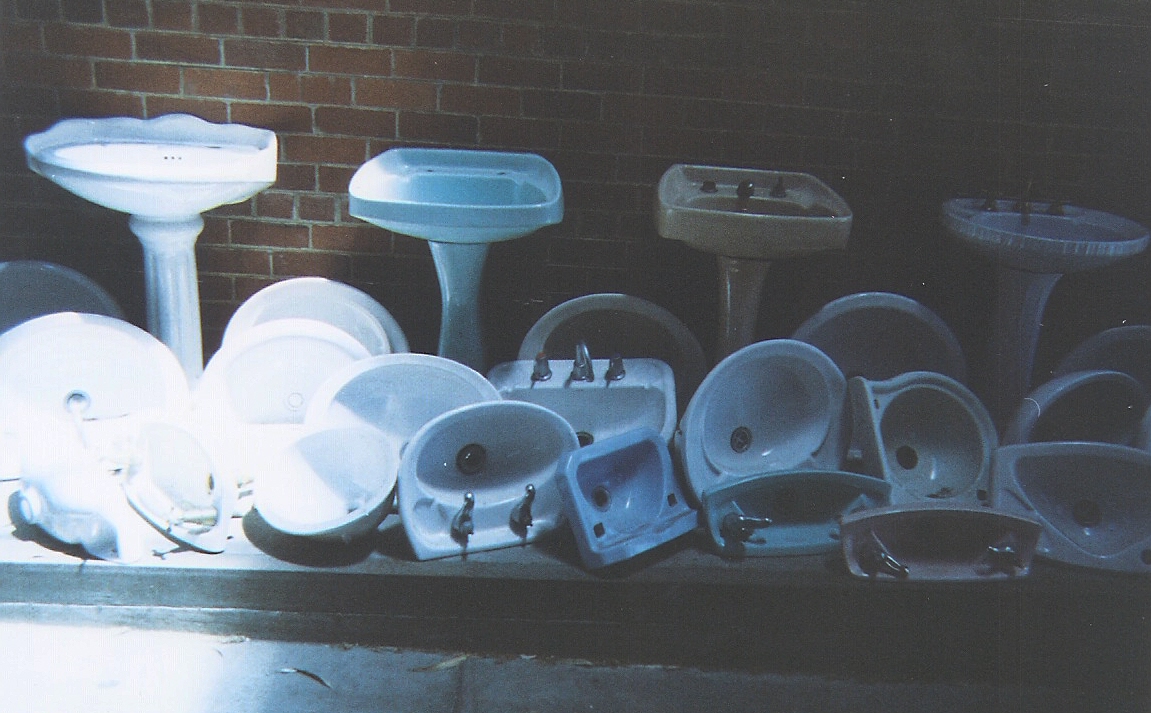In this outdoor photograph, a red brick wall with varying shades of orange and dark brown serves as the backdrop. Soft light from a diffuse source behind the camera and off to the left provides limited illumination, while the rest of the scene remains cloaked in shadow. The focal point is an assortment of porcelain sinks, with four standing upright in front of the wall. These sinks, each unique in design and color, range from a brilliant white one on the far left, supported by a vertical pillar, to shorter sinks in darker shades of brown and gray. The far-right structure has a rounded shape, reminiscent of a birdbath. Scattered haphazardly in front and on top of a concrete floor are at least 15 or 16 other sinks. These are disorganized, as if discarded, showcasing varying shapes and slight color variations from white to light blue-ish, contributing to the chaotic yet intriguing composition of the scene.